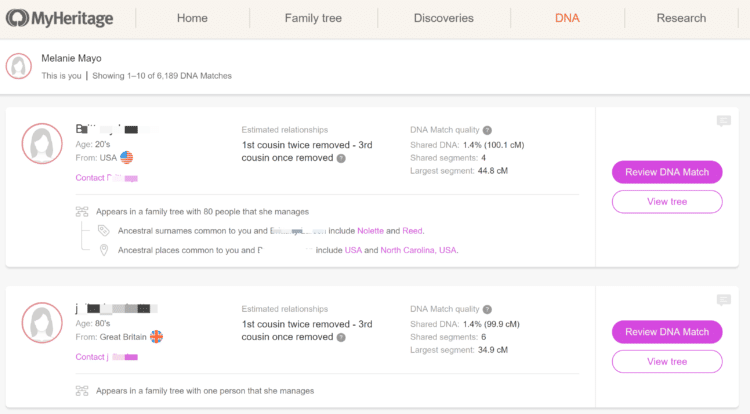This is a detailed screenshot from a webpage on MyHeritage. A beige banner at the top displays the MyHeritage logo on the left. The menu bar includes options labeled "Home," "Family Tree," "Discoveries," "DNA" (highlighted), "Research," followed by the user's name, "Melanie Mayo." Below, it indicates that Melanie is viewing DNA matches 1 through 10 out of a total of 6,189.

The first DNA match lists an individual, whose name is blurred out, aged in their 20s and residing in the USA. The estimated relationships are "first cousin twice removed" and "third cousin once removed." The DNA match quality is detailed as "shared DNA 1.4%, 100.1 cM, shared segments 4," with the largest segment being "44.8 cM." This individual appears in a family tree managed by them, which includes 8 people. Common ancestral surnames between Melanie and this individual are "NOLLETTE" and "REED." They share ancestral places in the "USA" and specifically "North Carolina, USA." The options "Review DNA match" and "View tree" are available.

The second DNA match involves another individual, whose name is also blurred out, aged in their 80s and residing in Great Britain. The estimated relationships are "first cousin twice removed" and "third cousin once removed." Their DNA match quality is "shared DNA 1.4%, 99.9 cM, shared segments 6," with the largest segment being "34.9 cM." This person appears in a family tree managed by them, which includes one person. Similarly, there are options to "Review DNA match" and "View tree."